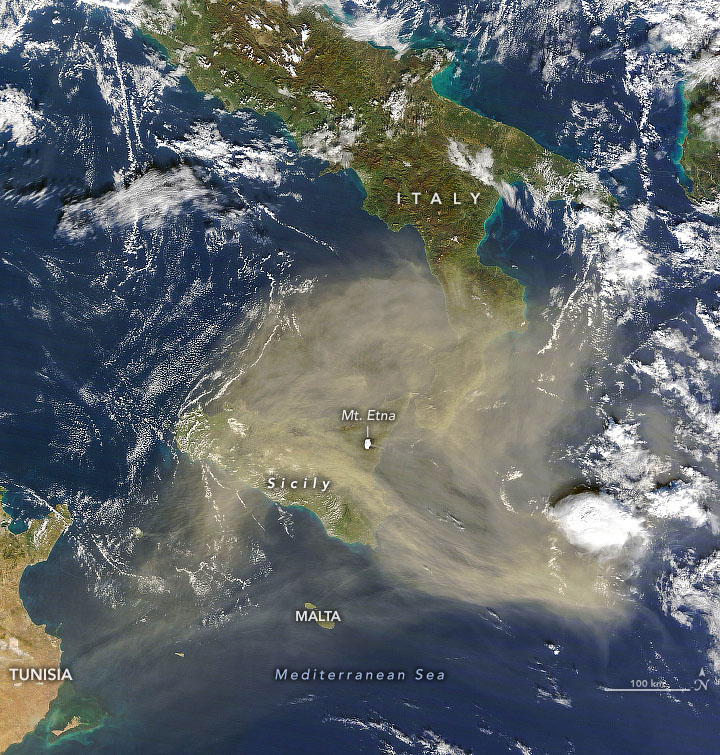This satellite image captures a detailed view of a segment of Earth, prominently featuring Italy and its surrounding regions. The image is essentially a high-resolution photograph of this part of the globe, not a traditional map, and is labeled for clarity. Distinctly, you can see blue areas representing the Mediterranean Sea, interspersed with white patches likely indicating clouds or snow. Alongside these, various green and brown land masses are visible. Key labels include Italy, Mount Etna, Sicily, Malta, Tunisia, and the Mediterranean Sea, with a small scale featuring 100 kilometers marked in the bottom right corner to provide a sense of distance. The prominent use of white text effectively points out and identifies these geographic locations, enhancing the educational value of the image.